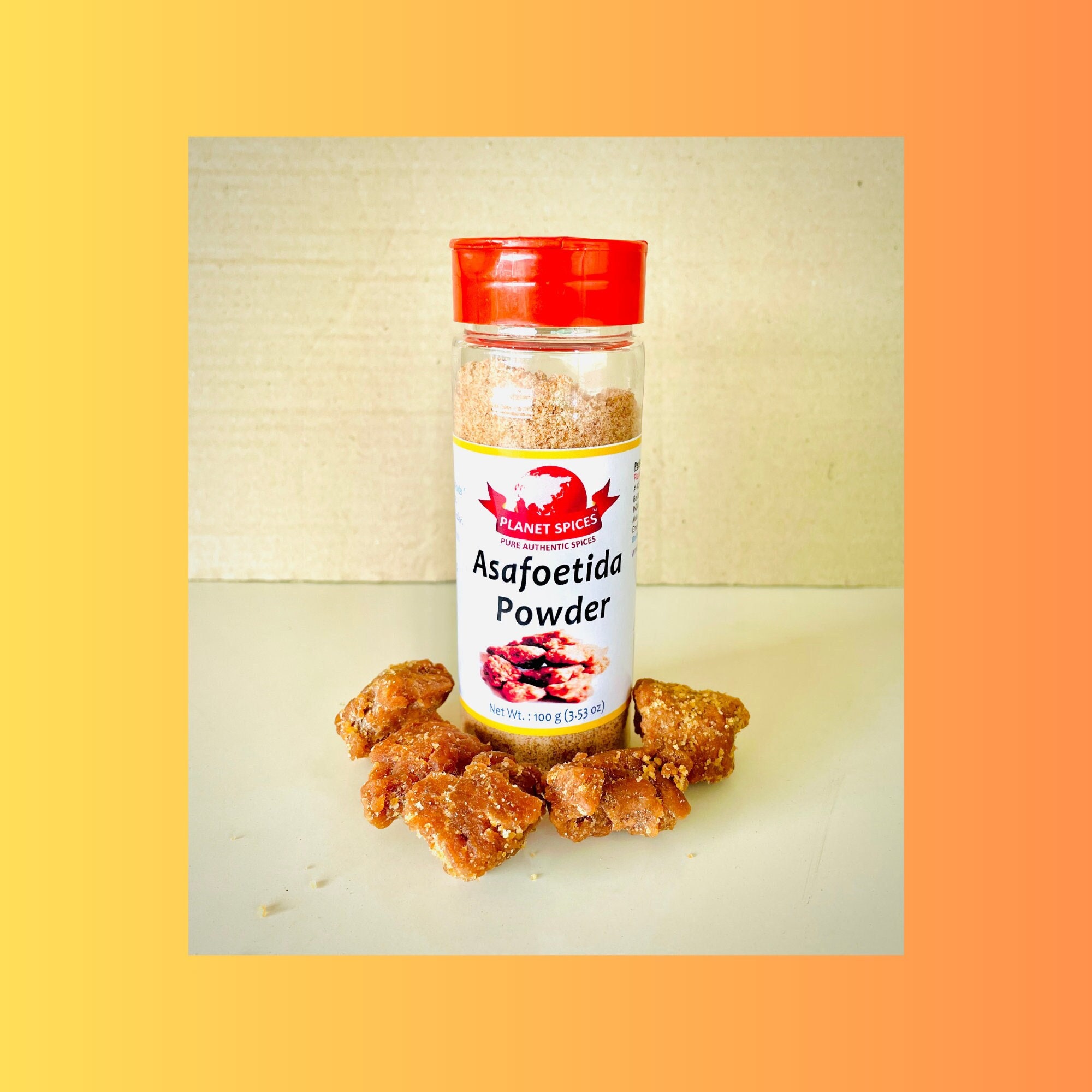The image is a detailed color photograph featuring a jar of Asafoetida powder from Planet Spices. The photograph is bordered by a gradient that starts yellow at the top left corner and transitions to orange as it moves to the right, becoming completely orange on the opposite side. The jar is clear, allowing visibility of the orangey-red tinted seasoning inside. It has a red cap, and the bottle is plastic. The white label with yellow borders at the top and bottom prominently features the Planet Spices logo, which consists of a red globe with a red banner declaring "Pure Authentic Spices." The label also displays images of the spice in its solid form and some food items garnished with the seasoning. The backdrop of the photograph is plain white, emphasizing the vibrant colors of the jar and its contents.